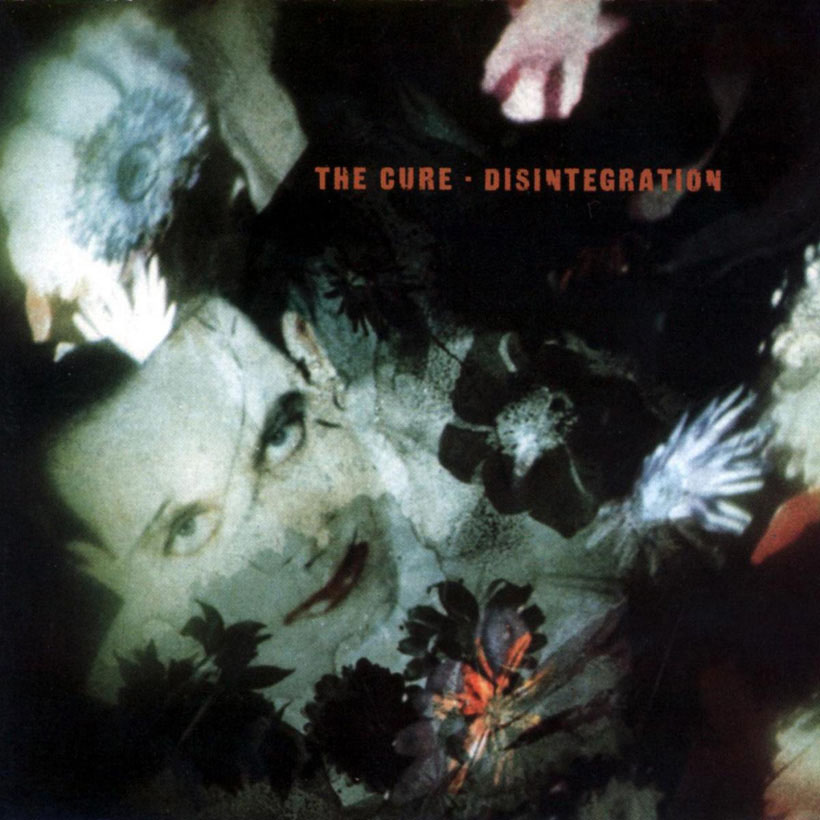The album cover for "Disintegration" by The Cure features an intricate and eclectic design. Prominently displayed in red lettering, the album’s title stretches across the top half of the cover. On the bottom left, the pale face of the lead singer, adorned with his signature dark black eyeshadow and dark red lipstick, looks upwards. Above him is a striking image of a solitary eye, further enhancing the cover's enigmatic feel. The entire composition sits against a dark background in hues of black, blue, and gray, interspersed with psychedelic elements including an array of flowers in shades of white, dark blue, and red. The artwork gives off a surreal, almost dreamlike atmosphere, with scattered plants accentuating the wild and fantastical theme.